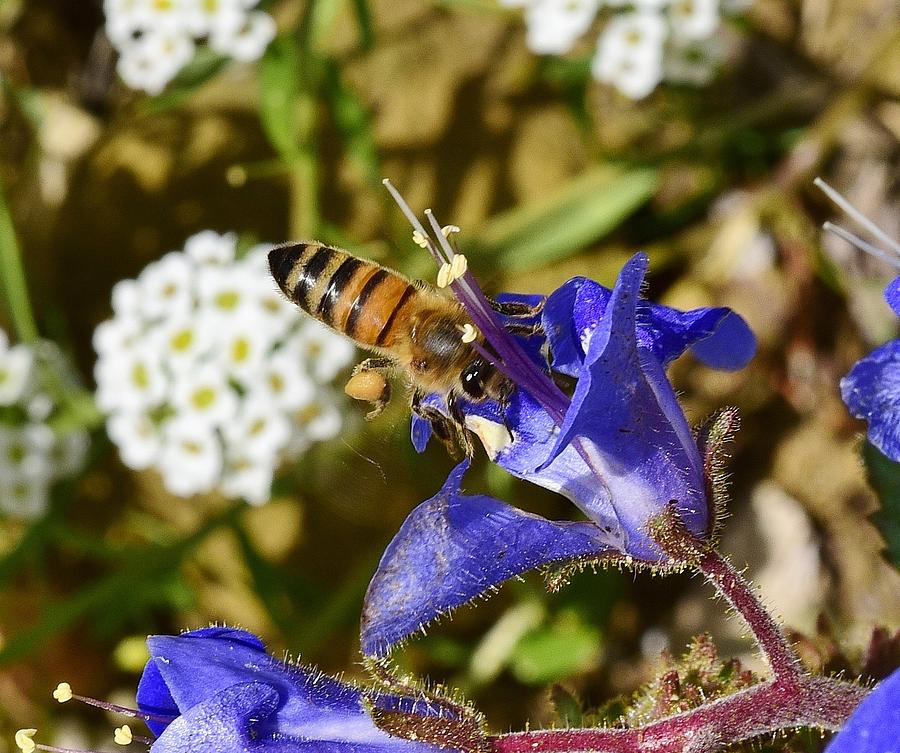This is a close-up photograph taken on a sunny day, capturing a detailed scene where a honeybee takes center stage, gathering nectar from a purple, cup-shaped flower that splits into four petals. The bee, with black and yellow stripes and fine hairs covering its thorax, is prominently perched on the petal. Surrounding the main flower are several other similar purple blossoms, all attached to a maroon-colored, slightly hairy stem. The background showcases a variety of white flowers with yellow centers, casting shadows on the crushed green blades of grass below, further emphasizing the bright daylight setting. The overall scene is rich with contrasting colors and textures, highlighting the intricate beauty of the bee and the flora.